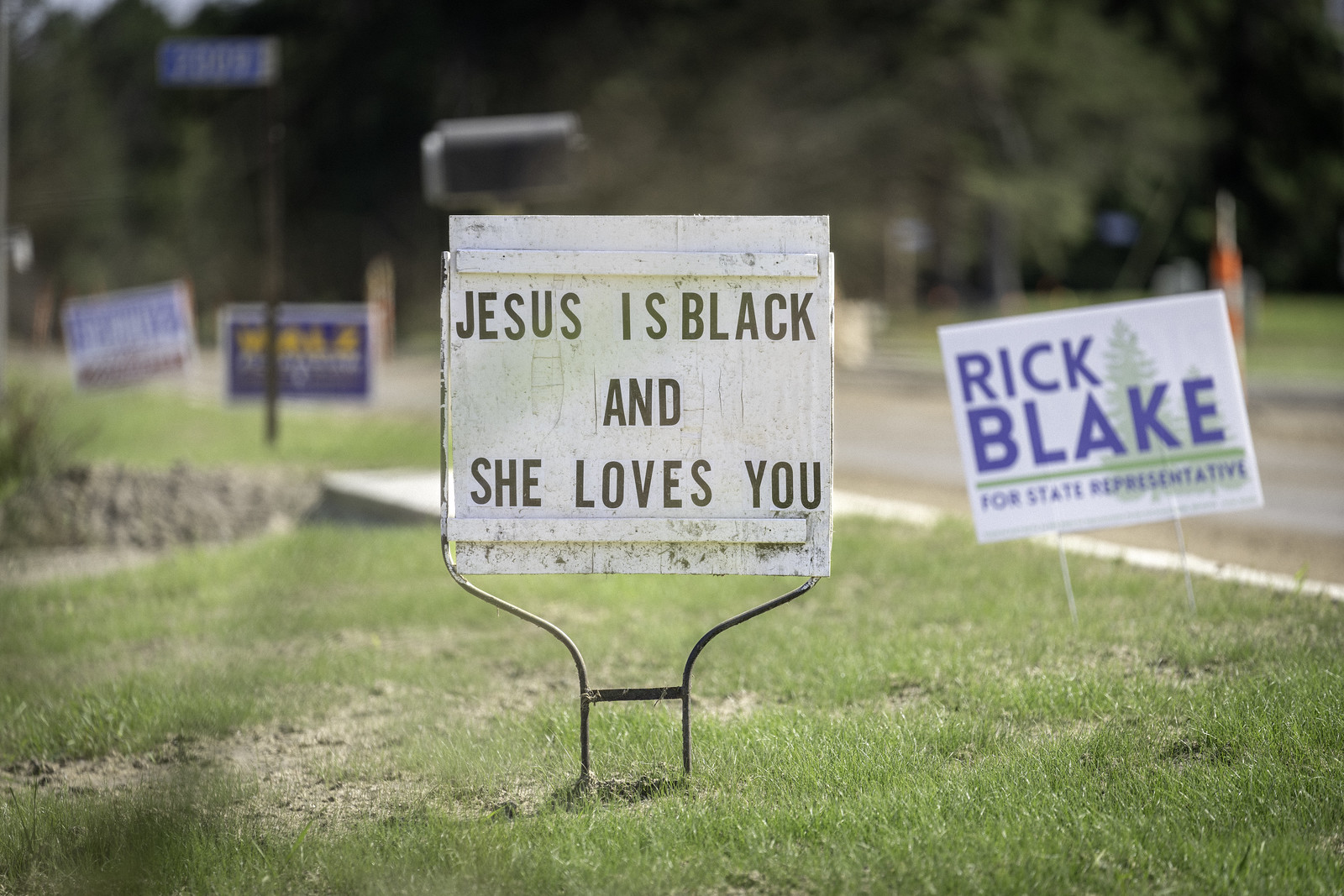This image showcases a yard sign placed on a patchy, green lawn with visible patches of dirt. The sign is supported by a metal base with decorative curls extending outward on both sides, connected by a horizontal bar, all painted black. The square sign itself, made of white-painted wood, features a message in black lettering stating, "Jesus is Black and She Loves You." The sign is framed by two horizontal wooden pieces at the top and bottom, enhancing its structural integrity and visual appeal.